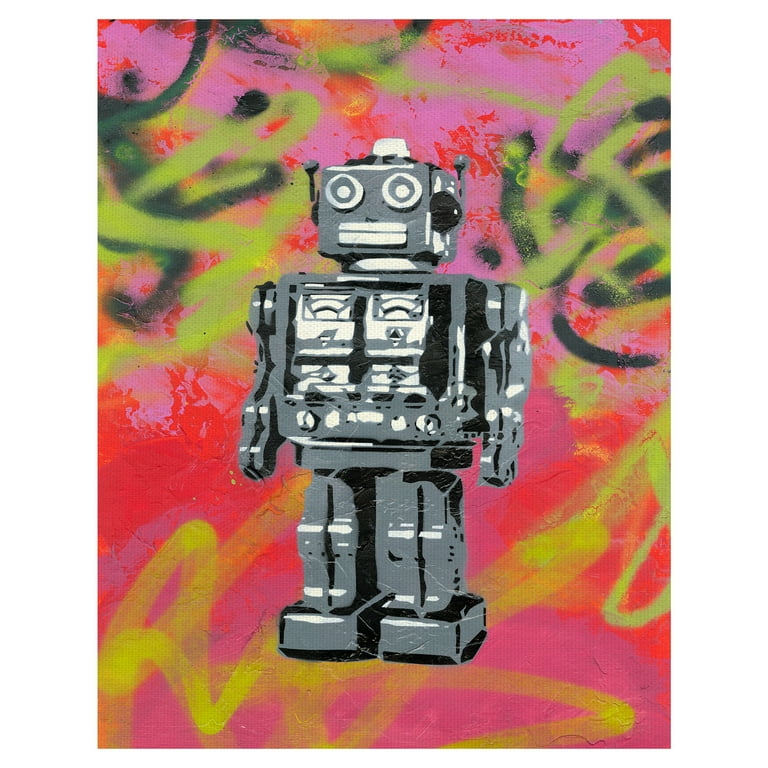The image captures a street art style painting reminiscent of Banksy, featuring a robot with a square head and body, rectangular legs on square feet, and arms at either side with hinged shoulders. The robot has a neutral expression, created using a mix of geometric shapes—white rectangular mouth, circular eyes with grey rings, and white centers—and a combination of circles, ellipses, and straight lines for the face. It has a light on top of its head and black knobs where its ears would be, along with antennae ending in knobs above the ears. The robot’s grey body is accented with white details, including gears in its belly and markings above its knees, ankles, and wrists that provide depth. The background is a vibrant compilation of graffiti in mixed colors—hot pink, neon yellow, deep pink, dark green, light green, red, and occasionally black— featuring abstract, free-flowing writing and unintelligible names. This chaotic backdrop contrasts sharply with the well-defined, gray robot standing slightly angled, making it the focal point of the image.